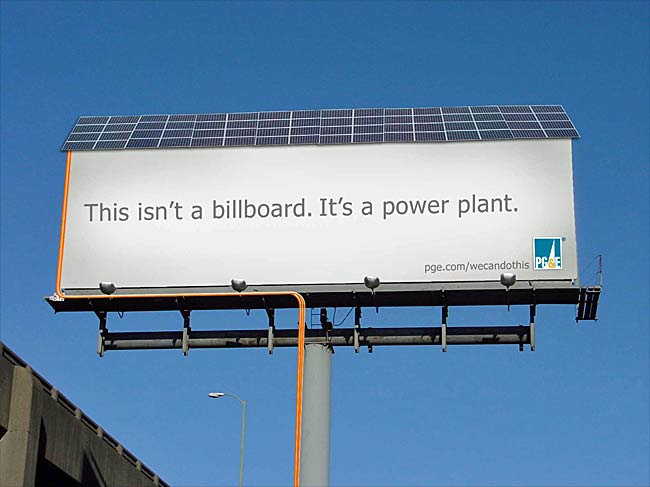The image features a white billboard topped with angled solar panels. A distinctive pink power line runs from these solar panels down towards the base, which is supported by a large, tubular gray pole connected to a horizontal beam. The billboard proudly displays a message in bold text: "This isn't a billboard, it's a power plant." In the bottom right corner of the billboard, the text reads "pge.com/WeCanDoThis". Adjacent to this text is a green square logo with the white letters "P, G, and E". The background sky is a solid medium blue, adding to the clean and modern aesthetic. In the lower center of the image, a street or building light on a post is visible, and a brown building occupies the lower left corner, providing context to the urban setting.